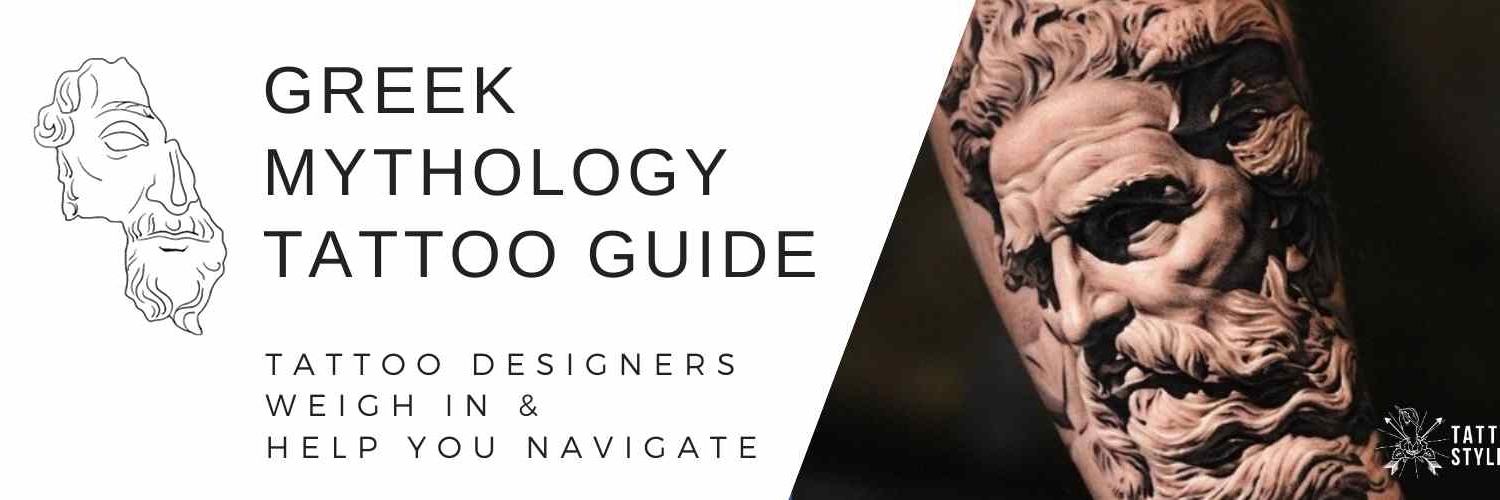The image is a black and white advertisement flyer featuring a detailed depiction of a Greek mythology tattoo. Dominated by the text "GREEK MYTHOLOGY TATTOO GUIDE" at the top in bold, large capital letters, it also includes the tagline "Tattoo Designers Weigh In and Help You Navigate" beneath it in smaller capital letters. The right side of the flyer showcases a tattoo of a man's face, resembling a stone statue, with intricate details such as long, flowing hair, a blowing beard, and a mustache. The face, with eyes open and a serious expression, appears to be carved and has a sculpted, stone-like quality. It's a lengthy tattoo, likely depicted on an arm. Adjacent to the main face image, a silhouette reveals only part of the head, showing the nose and right eye, enhancing the classical and mysterious aura of the design. The flyer effectively merges ancient mythological aesthetics with modern tattoo artistry to appeal to enthusiasts and potential clients.